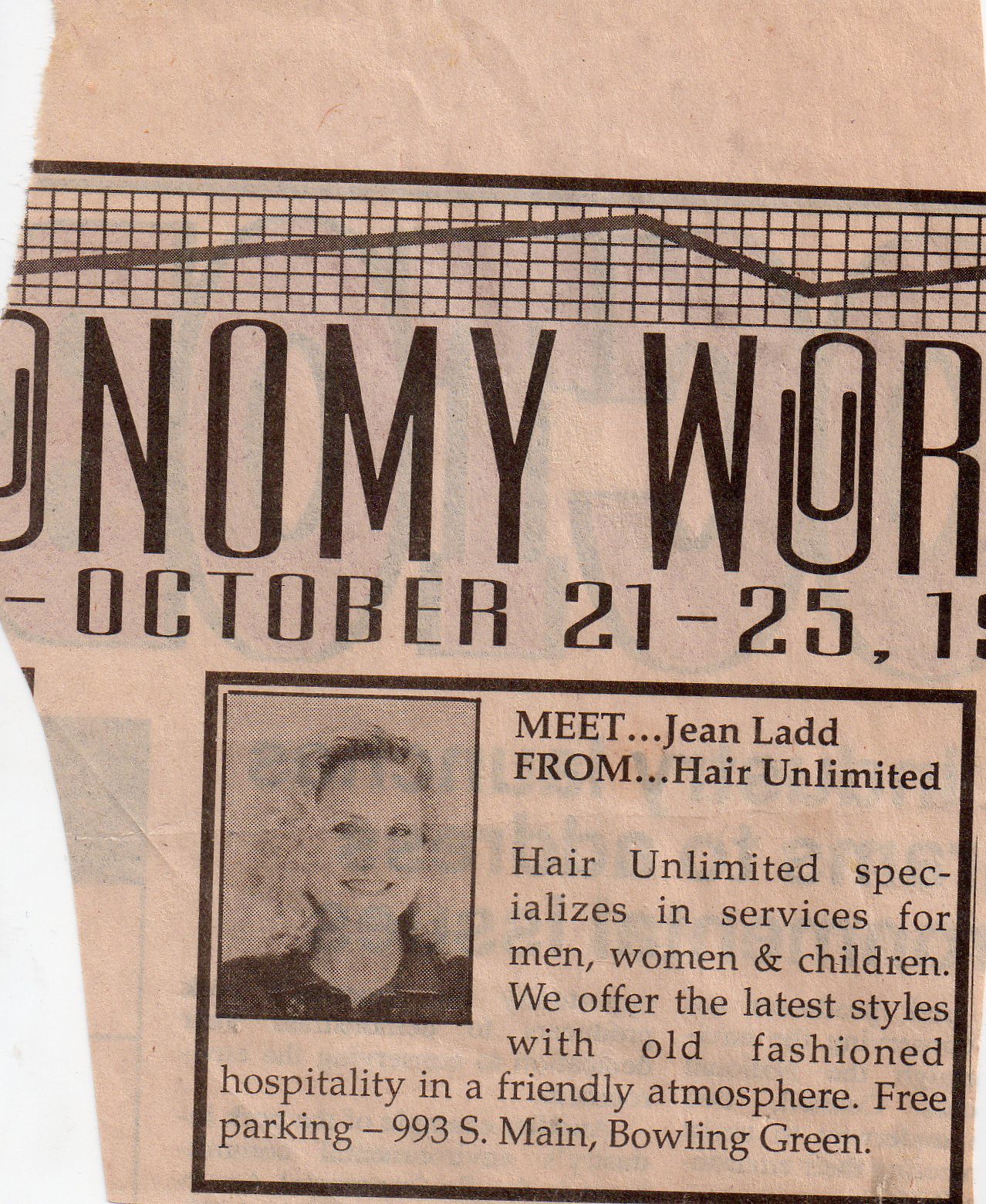This appears to be a clipping from an aged and slightly faded newspaper or magazine, indicated by its worn and folded condition. The visible part of the heading suggests it is from Economy World, although the text is partially cut off. The ad is dated October 21-25 from an unspecified year, but the design hints it might be from the 1980s. The centerpiece of the advertisement is a black square featuring a photo of a blonde, white woman accompanied by the text: "Meet Jean Ladd from Hair Unlimited."

Hair Unlimited is advertised as specializing in hair services for men, women, and children, offering the latest styles combined with old-fashioned hospitality in a friendly atmosphere. Free parking is available at 993 South Main, Bowling Green. The entire ad is enclosed within a bold black border. Above the photo, there appears to be a faded graph with a line extending up and down, contributing to the overall vintage appearance of the ad.